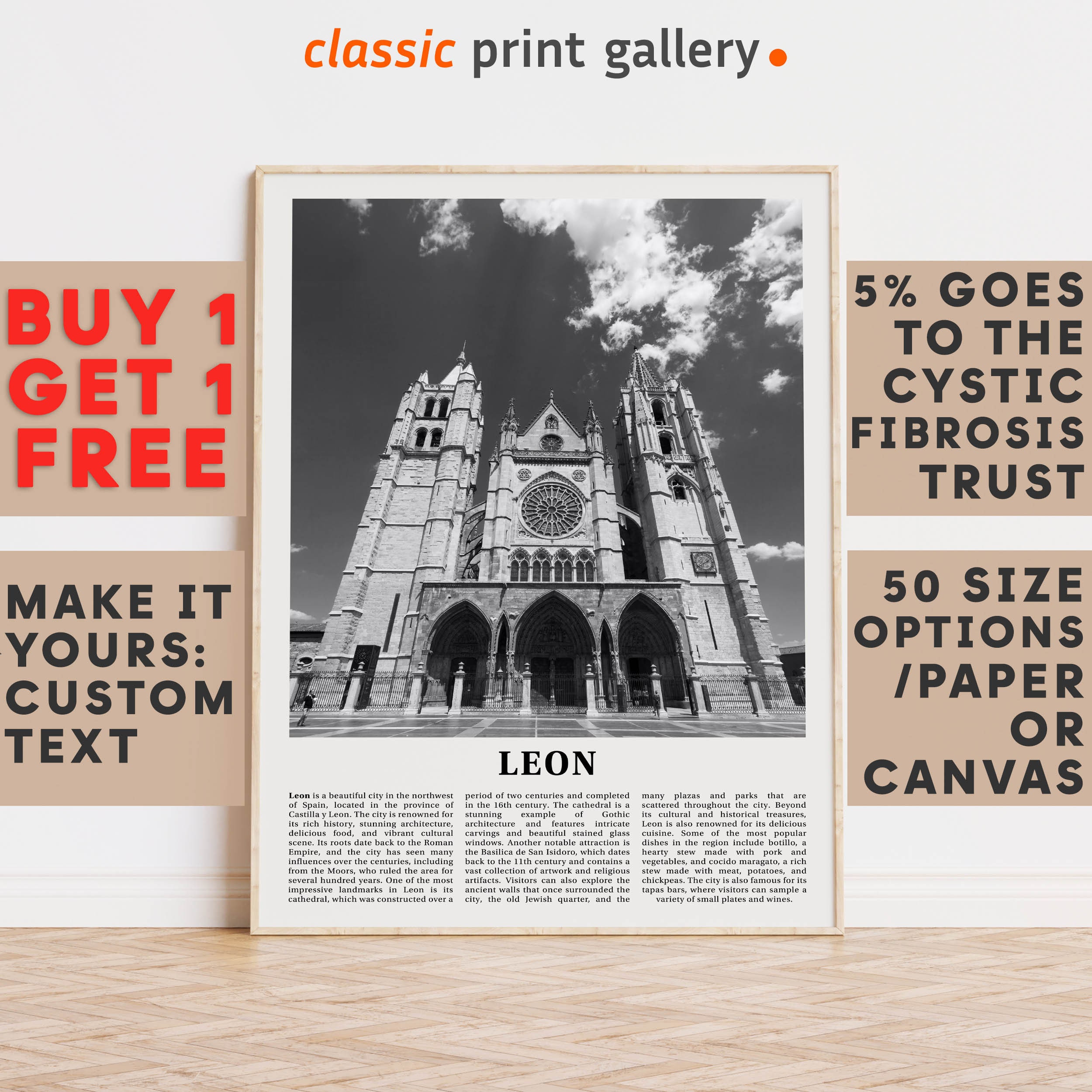A detailed image description:

The large, square photograph features a sign leaning against an off-white wall with a white baseboard at the bottom. The bottom section of the image displays a light-colored, zigzag-patterned wood tile floor. Central to the picture is a tall, framed poster with a thin natural wood border, leaning against the wall. The poster has a black and white photograph of an older building with two towers and three arched entranceways. Below the photo, the word "LEON" is printed in bold black capital letters, followed by three justified paragraphs about Leon, a city in northwest Spain, known for its rich history.

Above the picture, the wall displays the text "classic print gallery," with "classic" in orange italics and "print gallery" in dark gray. On either side of this title, there are tan-colored square signs. The top left square is red and reads "BUY ONE, GET ONE FREE" in all caps, while below it, another tan square states "MAKE IT YOURS. CUSTOM TEXT" in black, all caps. On the right, the upper tan square indicates "5% GOES TO THE CYSTIC FIBROSIS TRUST" in black, all caps, and the lower square notes "50 SIZE OPTIONS / PAPER OR CANVAS," also in black, all caps. This detailed composition suggests a promotional ad for a classic print gallery.